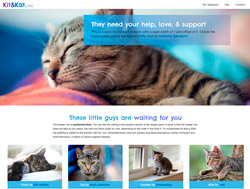This is a somewhat blurry screenshot of a website named "kitandkat.com," where both "Kit" and "Kat" are spelled with a "K." The website features a white background and prominently displays "kitandkat.com" on the top left, with "Kit" written in purple, "Kat" in blue, and ".com" in gray. On the top right, there is a navigation menu with three options, though the text is indecipherable due to the blur.

Below the navigation menu, there is a large, horizontal image of a young cat sleeping in what appears to be someone's lap. Overlaid on this image is a blue horizontal rectangle containing white text that reads, "They need your help, love, and support" in large letters. Directly below this image, some black text is present, but it is too blurry to read.

Following this section, there is another line in blue text that states, "These little guys are waiting for you." Beneath this line, there is a paragraph of black text, which is also unreadable due to the poor image quality.

At the bottom of the screenshot, there are four distinct navigation options, each accompanied by a picture of a cat. However, the text describing these navigation options is illegible because of the blur.